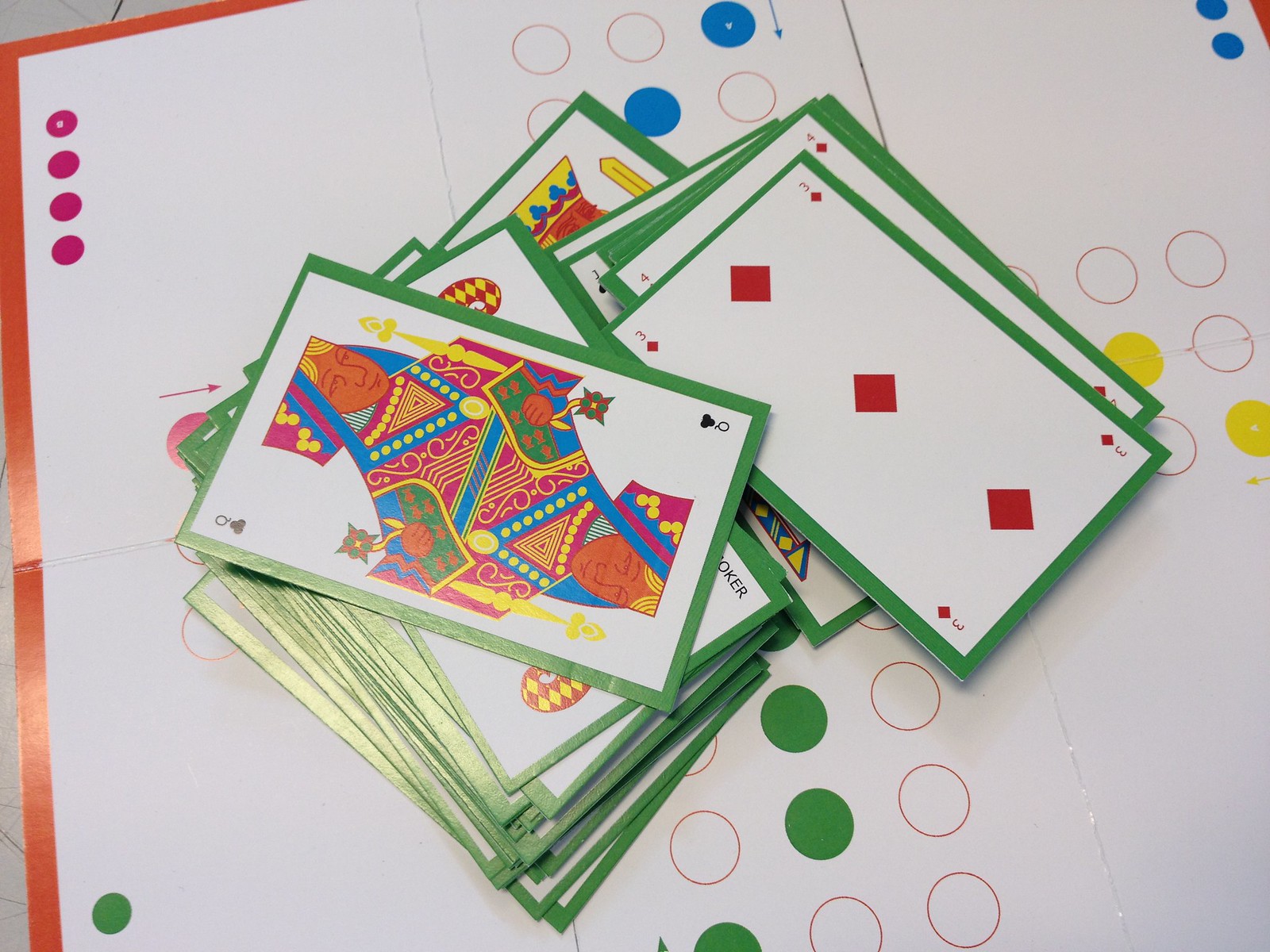This is a vibrant, color photograph featuring a white surface that serves as a game board. In the top left corner of the board, there are four vertical red circles, while near the bottom-right corner, a single green circle can be seen. The center of the game board is adorned with a pattern of multicolored circles, some of which are filled in with blue, green, and yellow, while others remain empty.

Dominating the scene are two messy stacks of large playing cards situated in the center of the image, obscuring a significant portion of the board underneath. The top card of the first stack is the Queen of Clubs, notable for its highly stylized and exceptionally vibrant illustration, featuring rich hues of yellow, blue, and red. Adjacent to this, the second stack has the Three of Diamonds face up, partially covering the Four of Diamonds underneath.

The photograph is devoid of any text or human presence, allowing the eye to focus entirely on the colorful and chaotic arrangement of cards and game board elements.